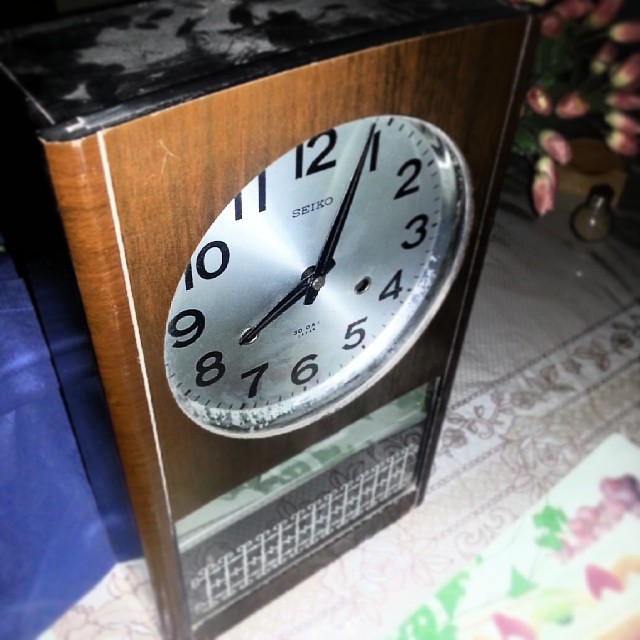This photograph showcases a Seiko mantel clock placed on a table draped with an off-white and brown floral-patterned cloth. The clock, with its rectangular shape, boasts a faux wood veneer exterior encasing a brushed stainless steel clock face. The black block-style numbers and the sleek black hour and minute hands stand out on the silver background. Above the hands, the brand name "Seiko" is distinctly printed in small block letters, with additional small writing visible below the hands, though it's not clear in this image. Positioned near the clock, but blurred in the background, there's a blue object and a vase of flowers, adding depth to the scene. The clock itself appears slightly dusty, suggesting it might need cleaning. The time displayed on the clock is set to 8:04.